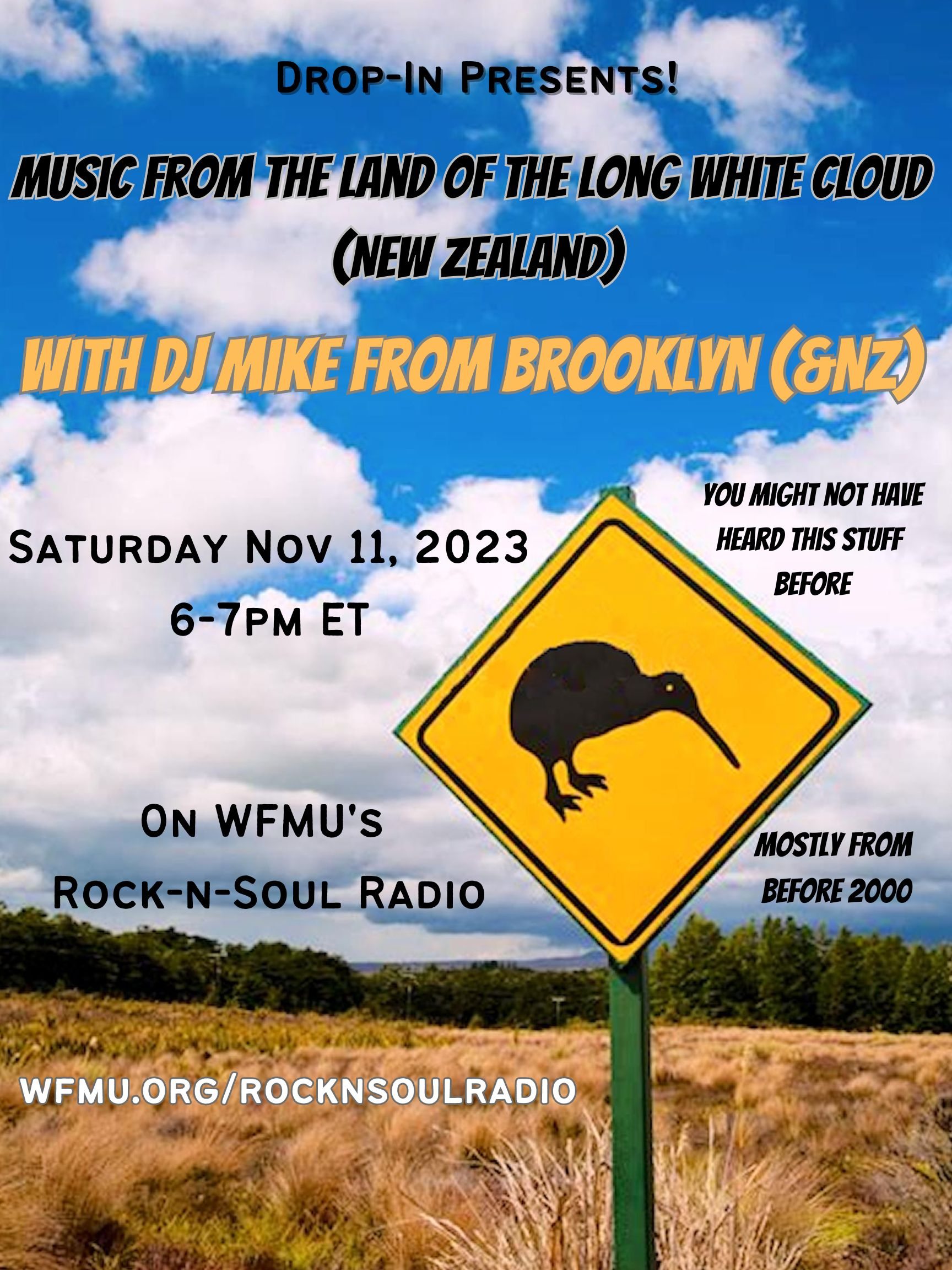The image is a promotional flyer for a radio event set against an outdoor scene with a blue sky dotted with white, fluffy clouds, and a landscape of golden grasses and green trees. A prominent feature is a green post with a diamond-shaped yellow caution sign depicting a black silhouette of a kiwi bird. 

The overlaid text reads in black: "Drop-In presents Music from the Land of the Long White Cloud (New Zealand)." Below that, in yellow, it states: "With DJ Mike from Brooklyn (and NZ)." The caption continues in black, providing the event details: "Saturday, November 11th, 2023, 6-7 PM ET" and "You might not have heard this stuff before." Further down, it mentions the broadcast will be on "WFMU's Rock and Soul Radio," adding that the music will be "mostly from before 2000." Finally, at the bottom in white text, the web address is given: "WFMU.org/RockandSoulRadio."